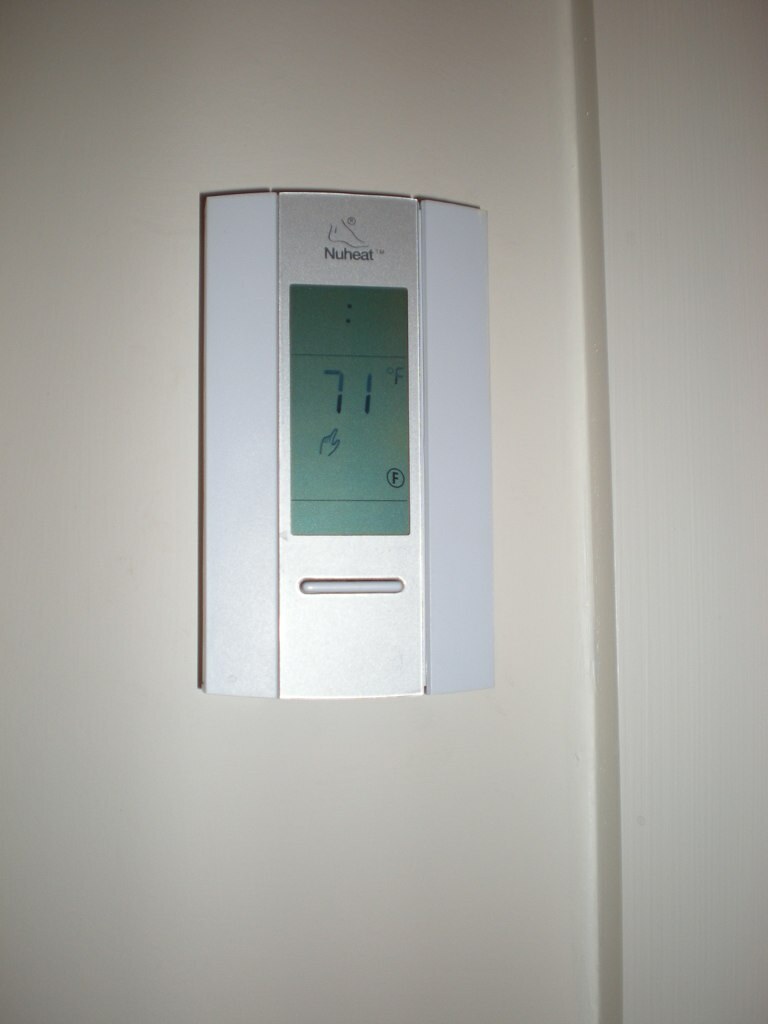This image captures a close-up of a modern thermostat interface mounted on a white wall. The central section of the thermostat is silver, while the outer panels feature a subtle gray hue. At the top of the display, the brand "NuHeat" is prominently displayed, indicating a high-tech heating system. Below the brand, a clear digital display shows the current temperature set at 71 degrees Fahrenheit, denoted by the "F" symbol. The interface also includes a hand icon pointing upwards, suggesting an increase in temperature or settings adjustment. Two colon dots in the middle of the screen add to the sleek, minimalist design. Overall, the composition and clarity of the thermostat provide a clean, user-friendly experience.